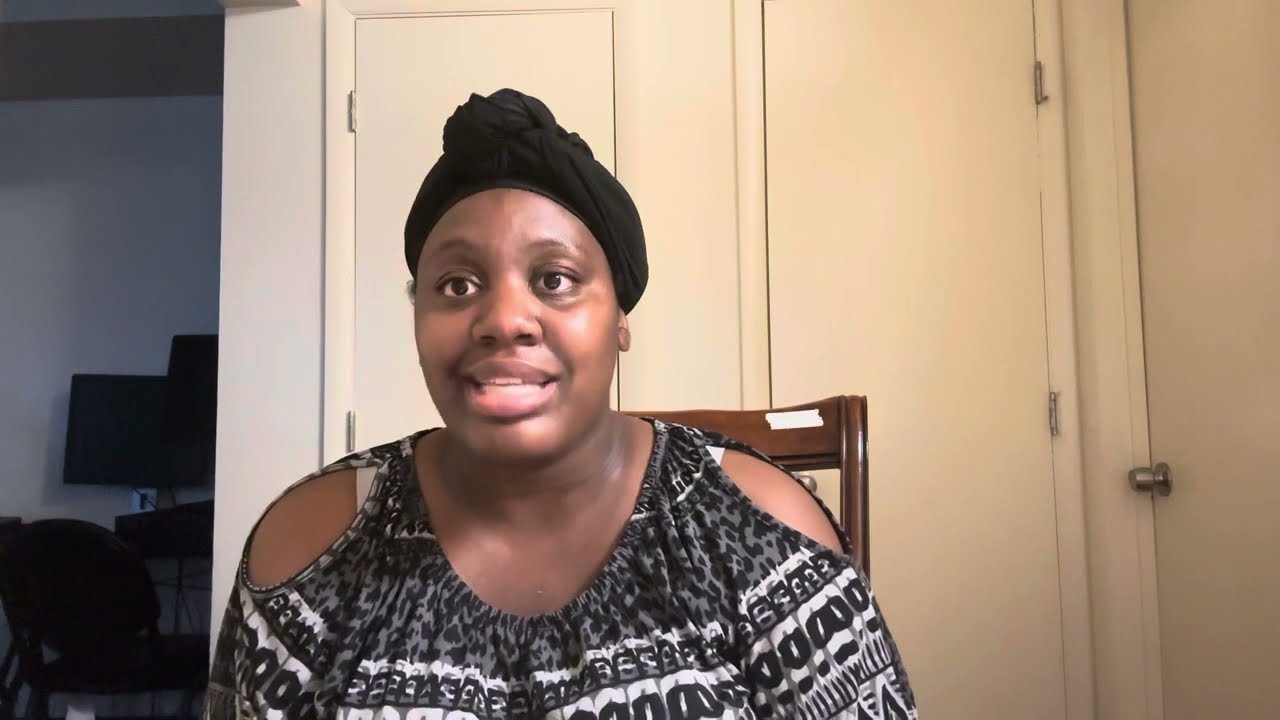The image features an African-American woman seated in a brown wooden chair, facing the camera and looking pleasantly engaged, possibly in the middle of explaining something. She has a black head wrap styled atop her head, and she's wearing a black and white patterned peasant top with shoulder cut-outs. The indoor setting includes three doors behind her; two narrow doors likely leading to storage closets, and a third door with a visible doorknob on the right. Behind her right shoulder, an open door reveals a dimly lit room with a TV, chair, and table. The walls in the background are a mix of white and tan hues. She has no visible jewelry or glasses.